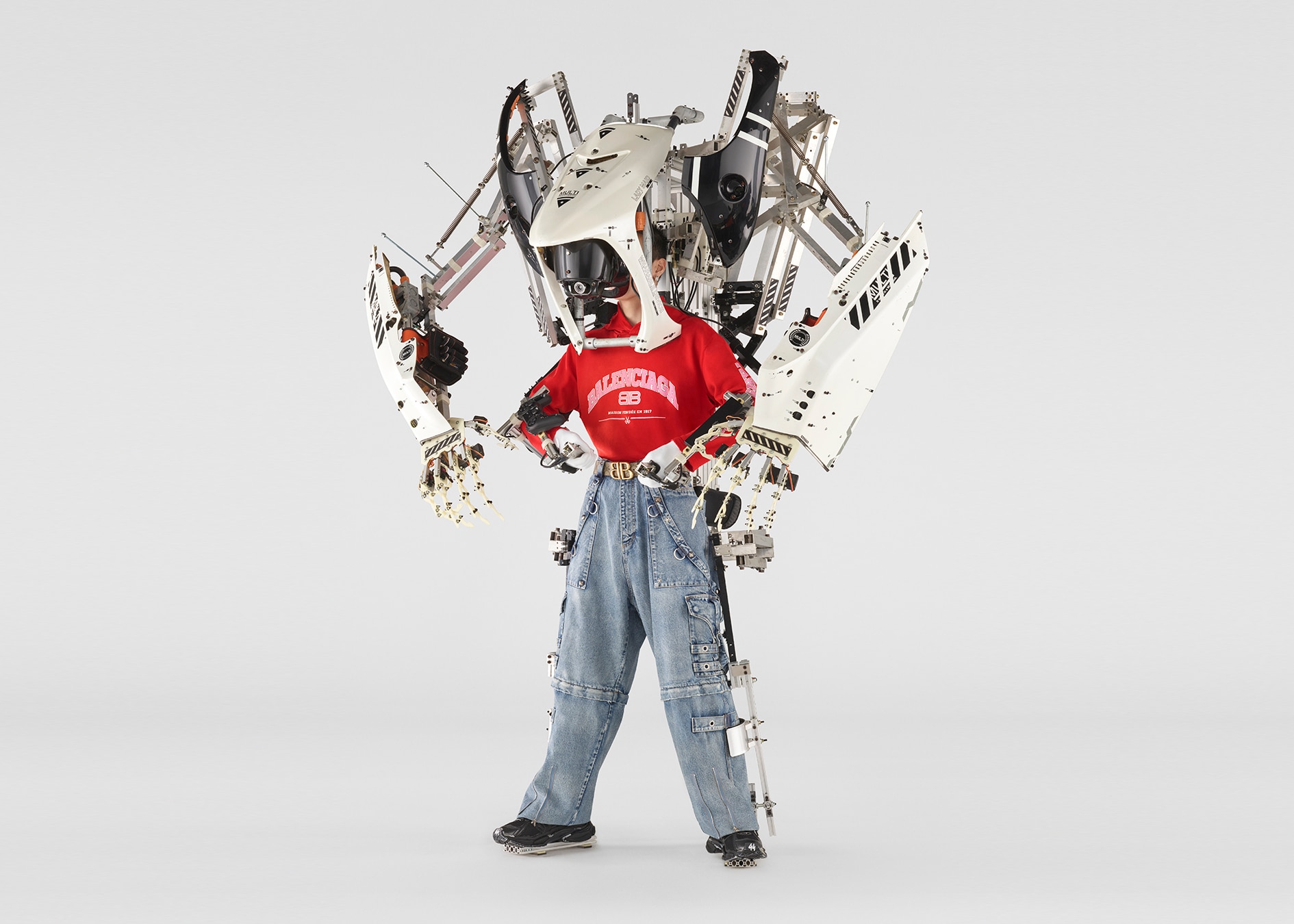The photograph depicts a man standing vertically against a plain white background, adorned in a red T-shirt, blue jeans, and black shoes. He is equipped with an elaborate and heavy-looking white exoskeleton, which is designed to enhance his physical strength and mobility. The exoskeleton features black lettering and trim, and encompasses various components including massive robotic arms, a faceplate hanging down in front of the man's face possibly integrated with vision aids, and a large harness secured around his waist, shoulders, and legs. The exoskeleton arms are mounted on a rail system that extends to the back, allowing for full range of movement. Additionally, cameras are visible on the uprights of the arms, and a heavy helmet-like apparatus appears to balance the weight of the structure, ensuring stability and support. The overall scene highlights the advanced technology of the exoskeleton, emphasizing its robust design and functional implementation in augmenting human capabilities.